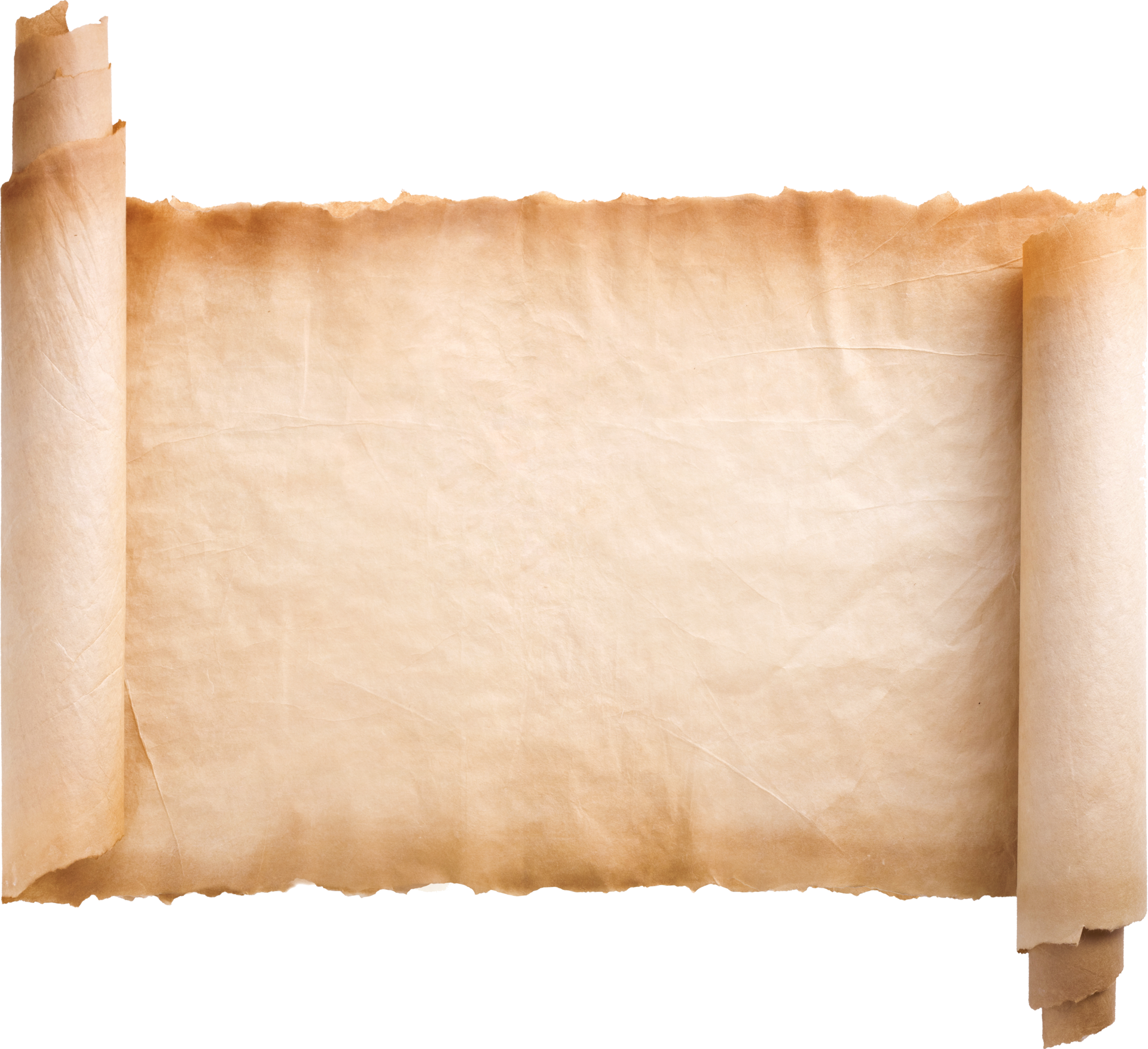This is a highly detailed, photorealistic image of a weathered, ivory scroll with frayed, browned, and almost burnt-looking edges that add a distinguished, aged aesthetic. The scroll is centered against a pure white, transparent background. Both ends of the scroll are rolled up, with the left and right sides creating prominent scroll-like rolls, while the middle section unfurls and lies flat. The surface of the parchment is marred with numerous wrinkles and creases, giving it a textured and rustic appearance. The paper itself is completely blank with no text or markings to indicate its age or origin.